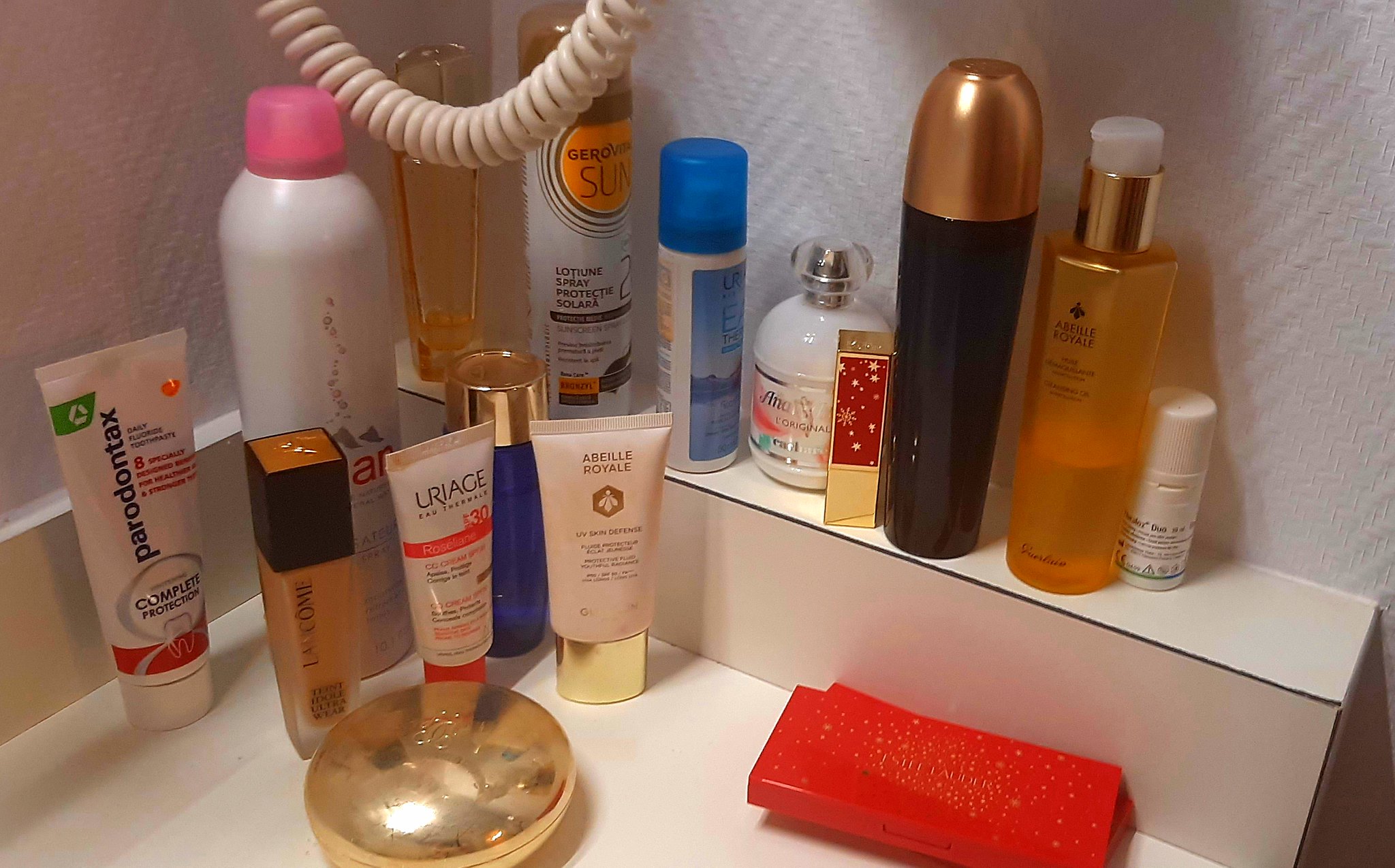The image captures a small corner of a bathroom showcasing a neatly arranged, compact ledge functioning as a shelf. On this shelf, a variety of beauty products are meticulously placed, creating a colorful and practical display. The assortment includes various ointments, lotions, and makeup items, although their specific purposes are not entirely discernible. Noteworthy items include what appears to be a mousse hair product, a toothpaste tube, and a sunscreen can equipped with a spray top for easy application. The shelf also holds an assortment of wrinkle creams and various makeup products. Among these items stands a small red box, whose contents remain a mystery but are likely beauty-related. Additionally, a coiled cord dangles nearby, suggesting the presence of a plug-in device such as a hair dryer, poised for convenient use.